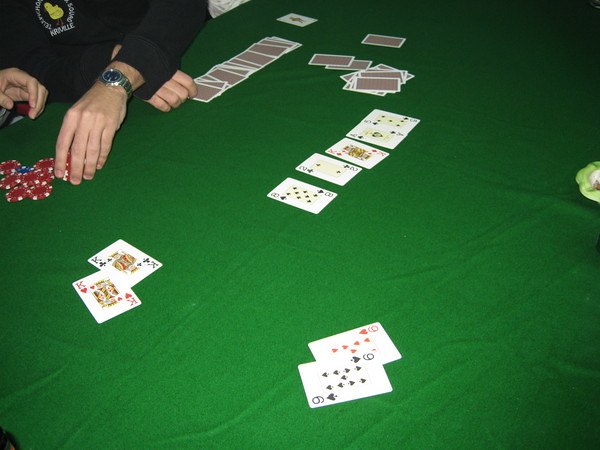In this picture, people are engaged in a card gambling game, captured vividly on a tabletop covered with green, fabric-like material that displays visible wrinkles and humps. Strewn across the table are numerous cards, with a specific line of cards running through the center. In the foreground, two stacks of two cards each are facing upwards, while in the background, several cards lie upside down. Before the man's hands, there is another line of upside-down cards. 

The man, who appears to be Caucasian, is dressed in a black, long-sleeved sweatshirt adorned with a small chick illustration and encircled by white text. A silver watch is visible on his wrist. One hand rests casually on the table near the cards, while his other hand is reaching out to grab several gambling coins, which include red ones and a single blue one. Additionally, another hand is extended towards him, indicating the presence of another player participating in the game.